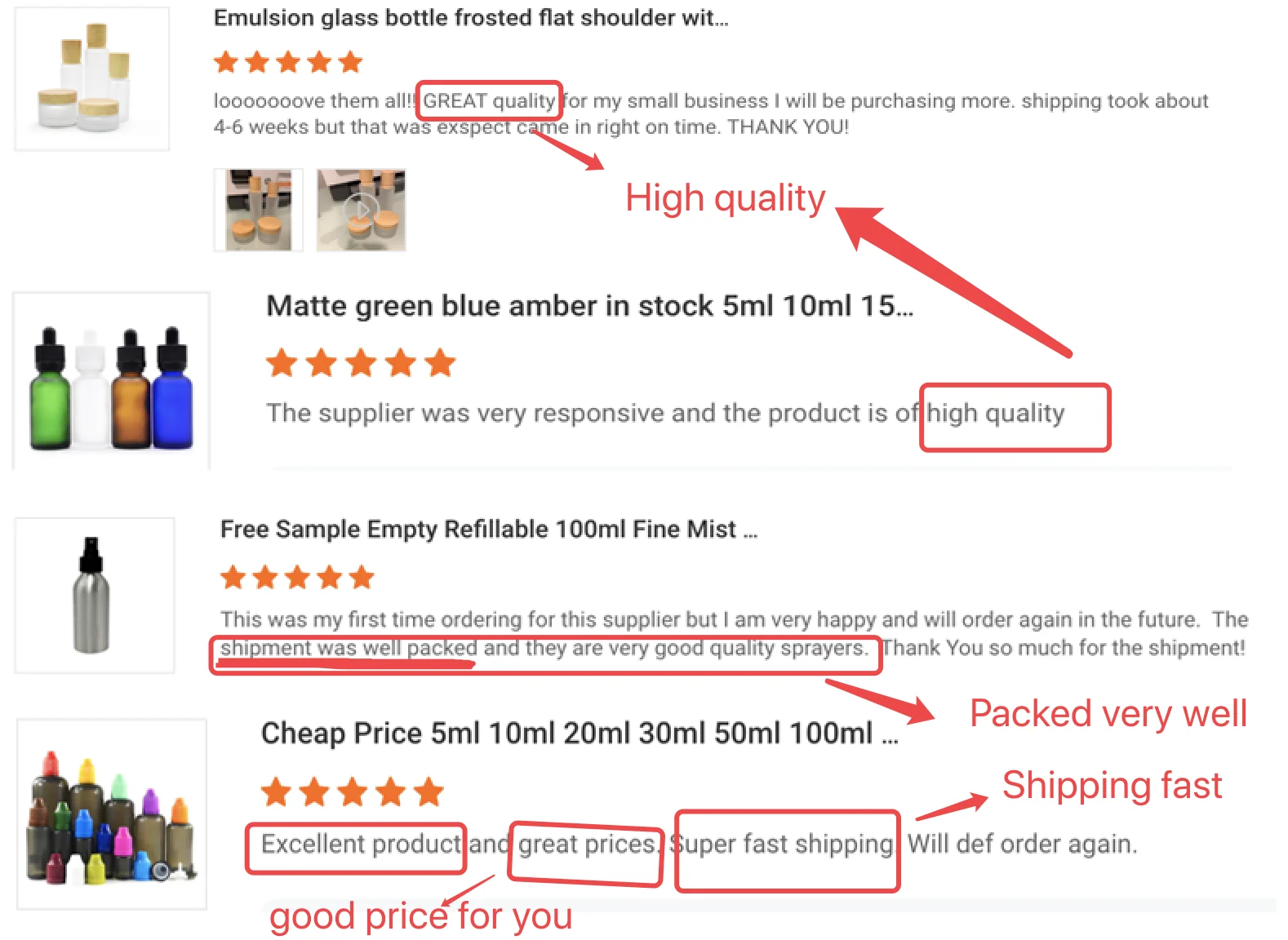The image features a detailed review and description of various frosted glass bottles with black text at the top reading "Emulsion Glass Bottle Frosted Flat Shoulder WIT...". On the left side, within a square, several different frosted bottles with brown tops are showcased. The review for these bottles gives them a perfect rating of 5 out of 5 stars and praises them with the comment, "Love them all."

Highlighted in a red box is the phrase, "Great Quality," followed by an arrow pointing downward to bold red text that reads, "High Quality." Below this, the available options are listed: matte green, blue, and amber bottles, each available in sizes of 5 milliliters, 10 milliliters, and 15 milliliters. 

Adjacent to these descriptions, there is another image showing the bottles in the mentioned colors, reiterating the 5 out of 5 stars rating. An additional note states, "The supplier was very responsive and the product is high quality," highlighted once more with another arrow and red square pointing to the phrase "High Quality."

Next, another review describes a free sample of an empty, refillable 100 milliliter fine mist spray bottle, accompanied by an image of a silver spray bottle. This product also receives a rating of 5 out of 5 stars. Within a square, underlined text highlights, "Shipment was well packed," with a red arrow pointing downward and the note, "Packed very well."

Lastly, the review covers "Cheap Price 5 Milliliter" bottles, again rated 5 out of 5 stars. It is highlighted within a red square that states, "Excellent product, great prices, super fast shipping."